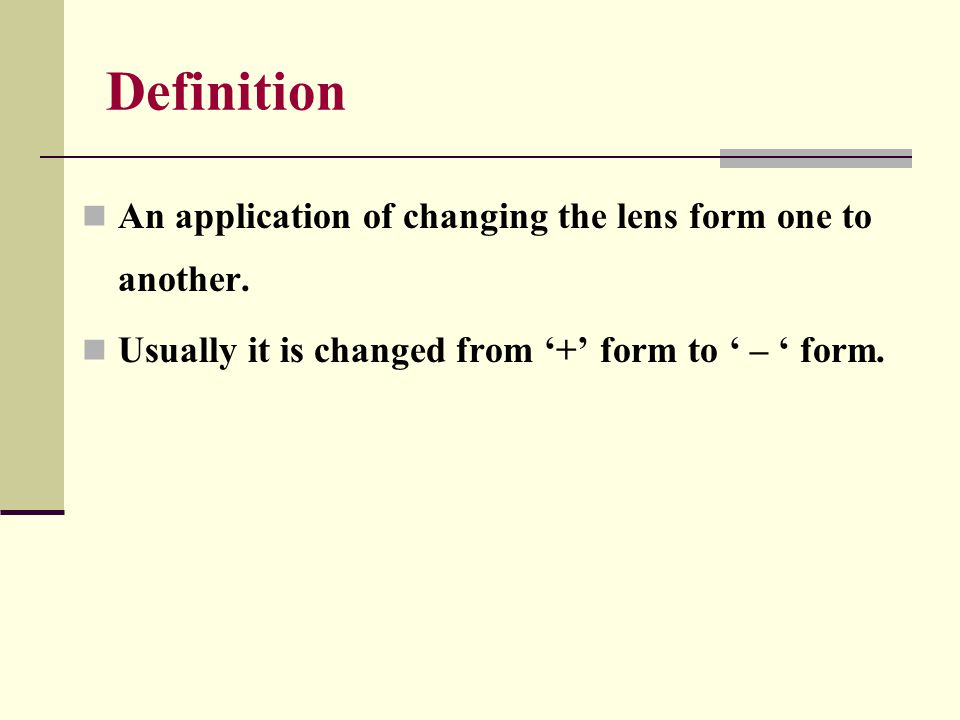The image features a slide with a title at the top that reads "Definition" in maroon, bolded Times New Roman font. Below the title, a dividing line splits the heading from the body of the slide. The slide's background is a light pale yellow color. There are two bullet points, denoted by small gray squares. The first bullet point reads, "an application of changing the lens from one to another." The second bullet point states, "usually it is changed from a plus form to a minus form," though the quotation marks around "minus" are incorrect, with two open quotation marks instead of a proper open and close set. Additionally, there is a large column on the side that is tan or brown in color, and another small gray box at the end of the slide's dividing line. The predominant colors in the slide are maroon for the heading, black for the text, and the pale yellow background, with accents of gray and tan/brown.